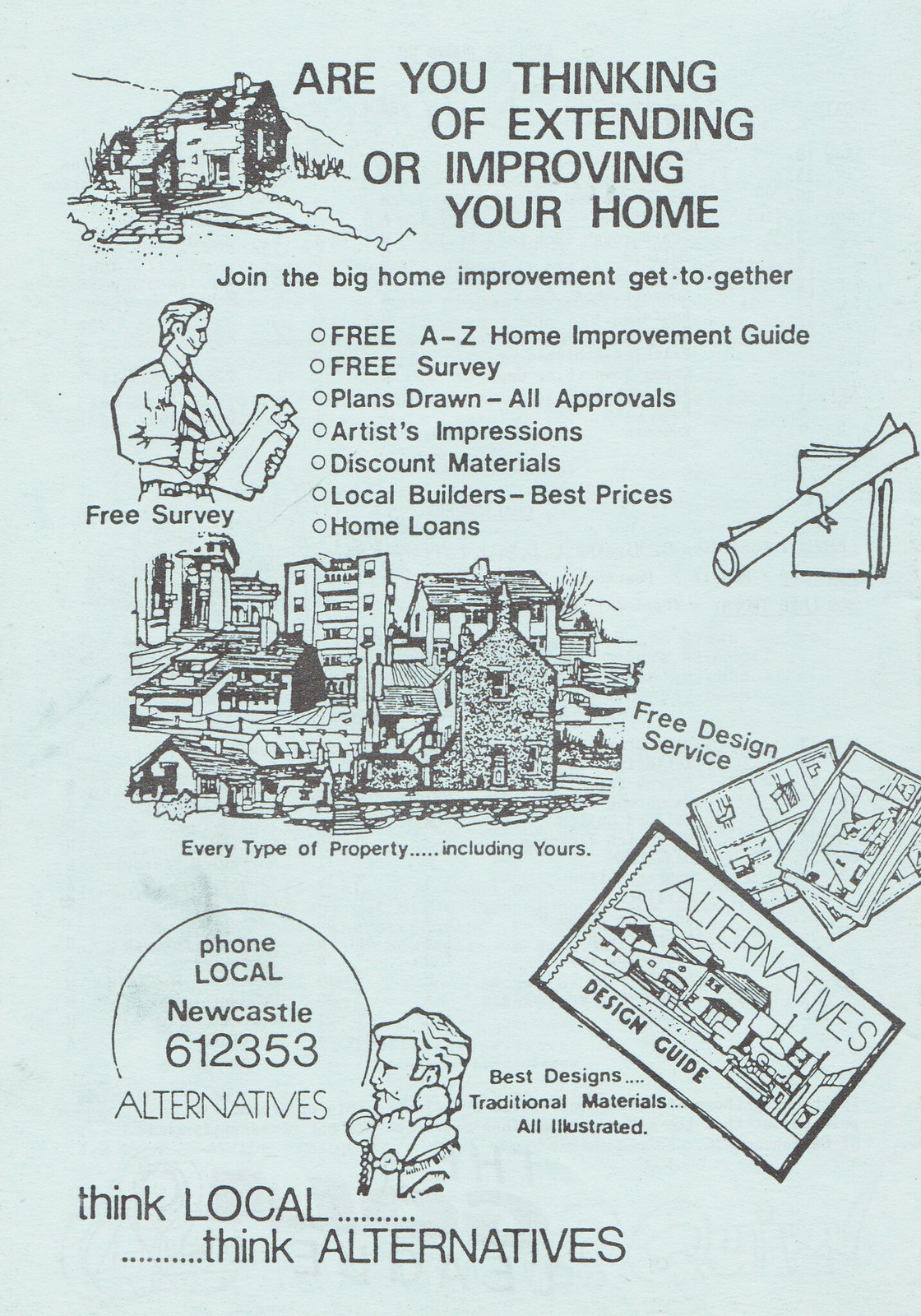The image is an old-looking, antique-style pamphlet on a light blue or light mint green background with black text. At the top left, there's a drawing of a house, and beside it, the title reads, "Are you thinking of extending or improving your home?" Directly beneath the title, another line invites readers to "Join the big home improvement get-together." The pamphlet advertises several offerings, such as a free home improvement guide, a free survey, plans drawn, all approvals, artist impressions, discount materials, local builders, best prices, and home loans.

Accompanied by a picture of a man standing, the text includes various images depicting more houses and buildings, as well as a rolled-up piece of paper which resembles a diploma scroll. Below these visuals, there's an artistic drawing of a suburban city skyline with a caption stating, "Every type of property, including yours." Towards the bottom, a slogan reads, "Think local, think alternatives,” and beside it, the pamphlet shows an illustration of a man's head with the phrase "Best Designs." The local contact number provided is "Newcastle 612-353." The layout of the text and images is somewhat scattered, but clearly aims to attract individuals interested in home improvement services provided by this company.